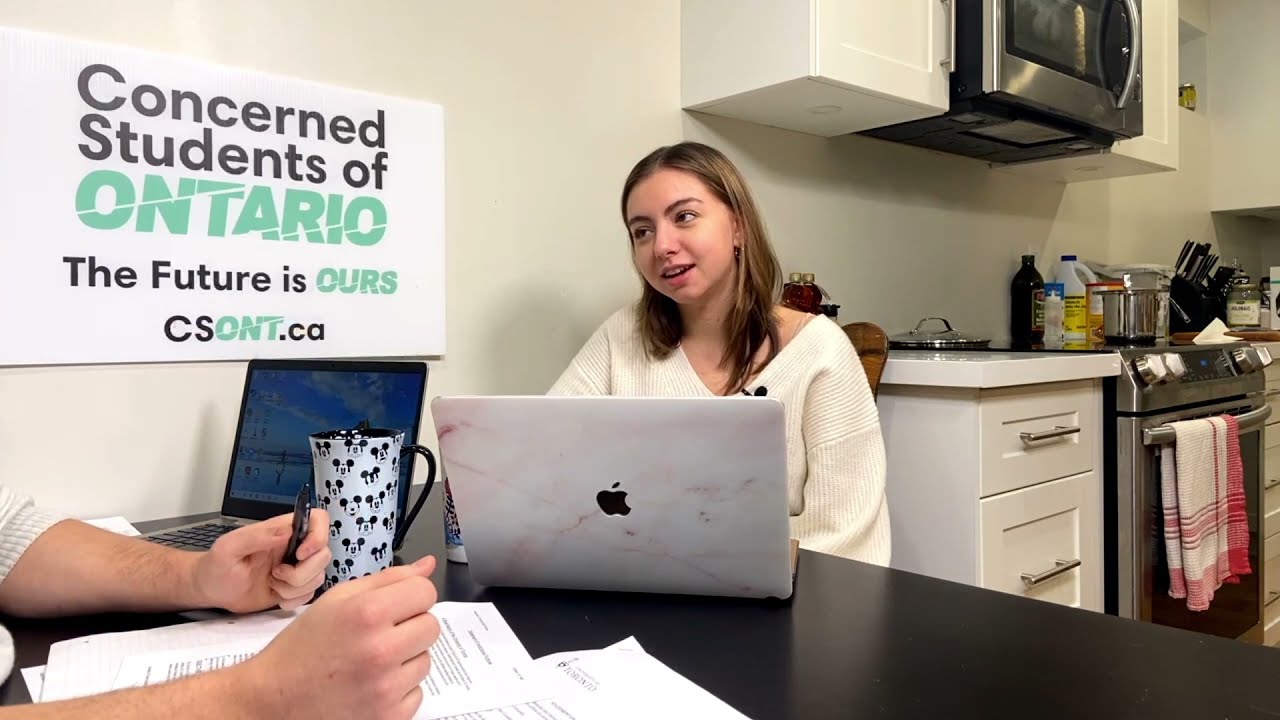In the image, two people are seated at a black table in a kitchen setting, appearing to work together or engage in a discussion, resembling an interview. On the left, the only visible part of the man are his hairy arms, suggesting he's male. He has various papers in front of him and a laptop to his left. Next to the laptop sits a white Mickey Mouse mug adorned with black-and-white faces of the iconic character. Opposite him is a young white woman with long brunette hair and brown eyebrows, wearing a white sweater and a clipped microphone. She's smiling at him while using her MacBook, identifiable by the visible Apple logo. A prominent sign on the wall beside her reads, “Concerned Students of Ontario. The Future is Ours,” followed by the website csont.ca, with selective text highlighted in green. The background reveals a kitchenette featuring a silver stove with a towel hanging from its handle, a microwave above it, white cabinets, and an assortment of bottles and cutlery scattered on the counter.